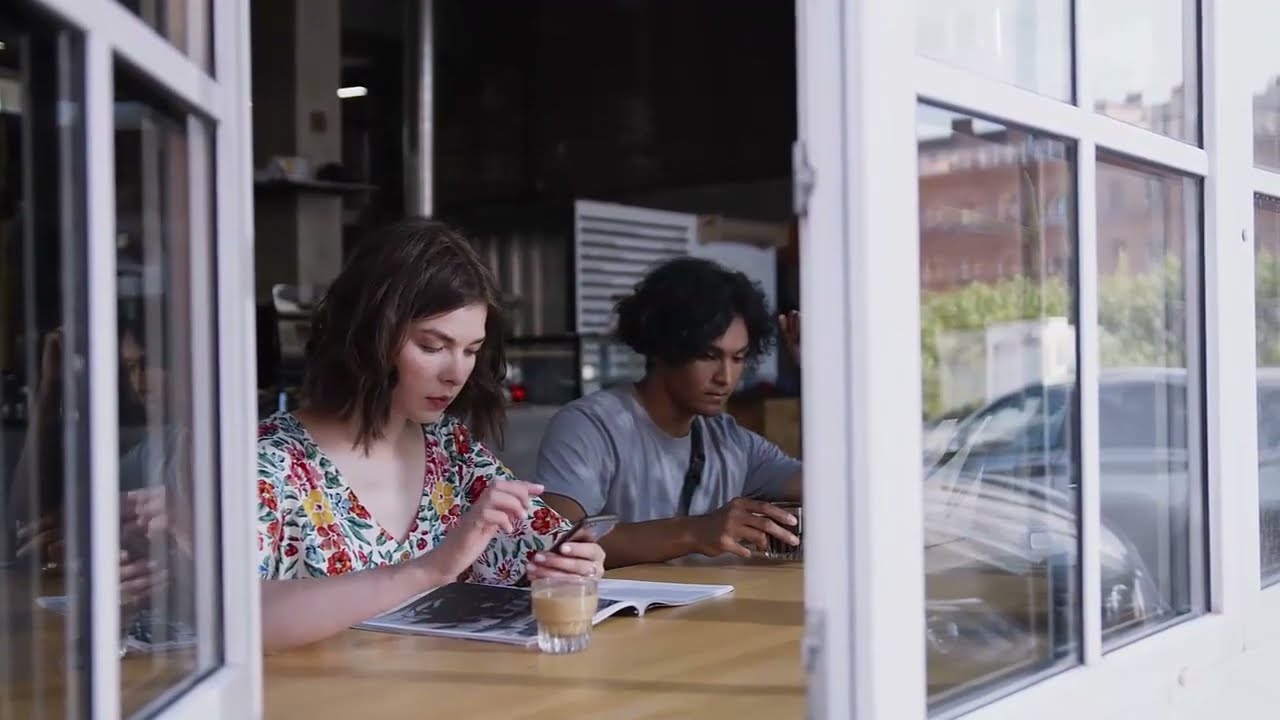This image captures a candid moment of a man and a woman sitting at a light beechwood table inside a coffee shop, viewed through an open window with white framing. The window on the left side is ajar, offering a clear sightline into the cozy interior. The woman, a Caucasian with long brown hair wearing a floral shirt with pink, red, and green leaf patterns, sits engrossed in her smartphone. In front of her lies a magazine and a glass cup of light brown coffee. Beside her is a darker-skinned man, possibly of Indian or Arabic descent, with long curly hair parted down the middle. He wears a gray shirt and holds a clear glass of black coffee. The background is tranquil, with no other patrons in sight, emphasizing the intimate setting of the scene.